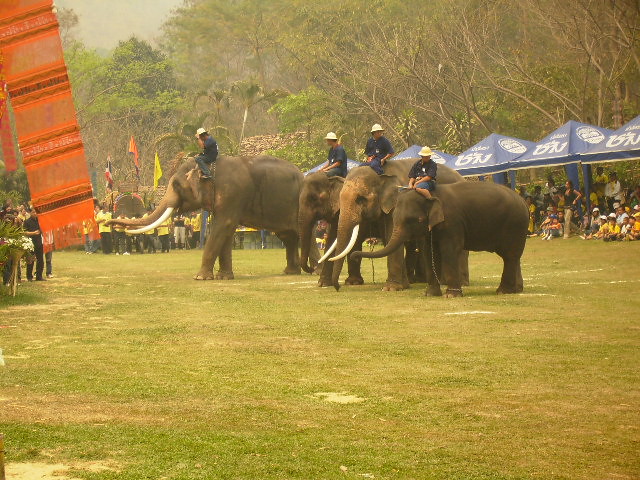This photograph captures an outdoor festival or event in what appears to be a southwestern Asian country, possibly Thailand. The scene is set in a grassy area surrounded by numerous trees. Dominating the foreground are four elephants, varying in size and color, with two possessing long ivory tusks. Each elephant is ridden by a man dressed in a blue shirt and white hat. The men, who seem to be of Asian descent, sit on the elephants without saddles, perched directly on their necks. 

In the upper left corner of the image, an orange contraption adorned with black stripes descends from the sky. Spectators are gathered around the scene, some standing and others sitting beneath blue, triangular event tents featuring non-English Asian script, which could be Thai. The tents presumably offer shelter, possibly from rain. The overall atmosphere of the event suggests a festive gathering, yet the image conveys a sense of neglect, with the elephants appearing sad and their legs chained, highlighting the tension between celebration and cruelty.